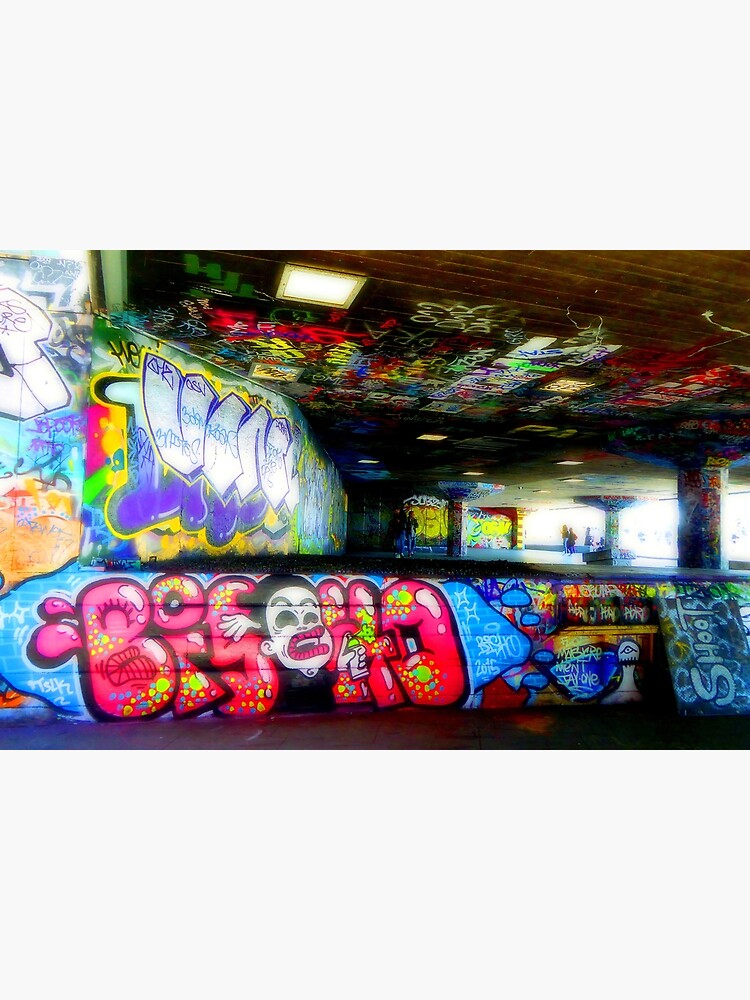The photograph captures a vividly colorful, underground parking structure or public space that serves as a canvas for a plethora of graffiti. The scene is drenched in neon hues, including purples, pinks, greens, whites, yellows, and more, each in their brightest possible versions. Graffiti covers nearly every surface: the ceiling, column posts, lower walls, and walls in the background. The artwork includes both illegible graffiti script and more discernible characters, such as a notable figure with black hair, a white face, bright pink lips, and a black dress, seen spraying green paint. The word "shoot" is visible on the right side of the image. The indoor area features multiple pillars and functional lighting, suggesting the space is operational. A group of people is visible in the background, adding life to the scene, which looks both eerie and captivating due to the mixture of the vibrant graffiti and the surrounding architecture. The sun shines through openings, adding a touch of natural light to the vividly decorated environment, reminiscent of an outdoor stage.